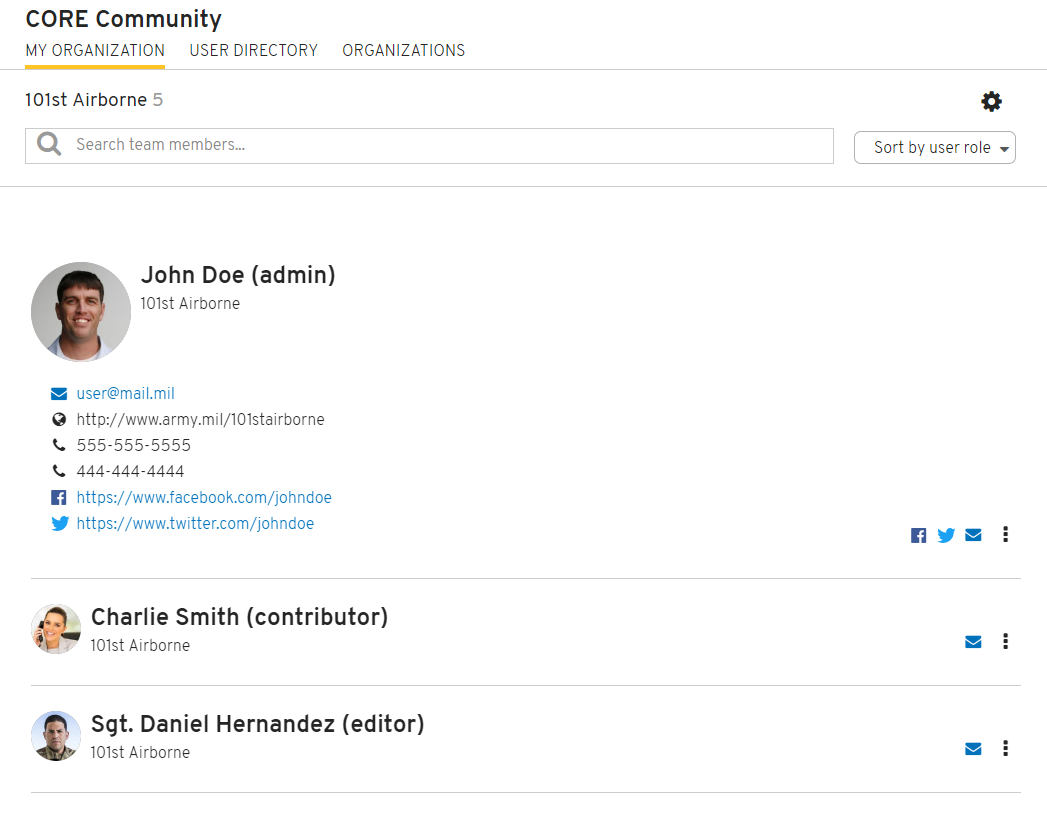In the upper left corner of the image, the phrase "Core Community" is prominently displayed. Beneath this, the words "My Organization" are underlined in yellow. To the right of this is the section labeled "User Directory," and further to the right is the section labeled "Organizations." 

Moving downward, the text "101 First Airborne" is visible, followed by a magnifying glass icon inside a long search bar. To the right of this search bar is a settings wheel icon. Below this, there is an option labeled "Sort by User Role."

Further down, an image showcases a man's face inside a circular frame; he has short brown hair and is smiling. Next to his image, the name "John Doe" is displayed with the designation "Admin" in parentheses. Below his name, it states "101 First Airborne." Adjacent to this are symbols and links corresponding to various contact methods: an envelope icon with the email "user@mail.mil," "army.mil," a Facebook link "facebook.com/JohnDoe," and a Twitter link "twitter.com/JohnDoe." A long line separates this profile from the next.

The next profile picture features a woman holding a telephone and smiling. The name "Charlie Smith" appears alongside her image, with "Contributor" noted in parentheses. Below her name, the unit "101 First Airborne" is repeated. Further down, another profile lists "Sergeant Daniel Hernandez" with the role "Editor" in parentheses, also associated with "101 First Airborne."